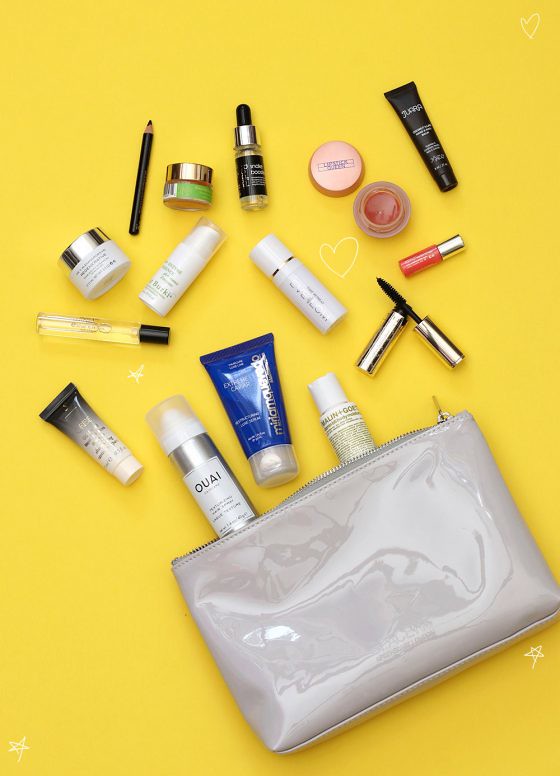The image features a vibrant yellow background with a prominent yellow rectangle and a small five-pointed star located in the bottom left corner. Spilled across this background are 17 variously arranged makeup items, suggesting a burst of cosmetic chaos.

On the leftmost side, there's a tube displaying a black-to-white gradient. Next to it is a sleek, silver tube branded with "WEI". To the right, a dark blue tube with a silver cap stands out conspicuously. Centrally placed at the bottom of the image is a shiny, reflective silver makeup bag. Resting above this bag is a white tube adorned with a white tab, though the text on it remains illegible.

Further detailing includes an open eyeliner set, presenting a silver tube with a slender black brush protruding from it and the detached cap situated to the left. Above this eyeliner, a petite pink bottle with a silver cap catches the eye, alongside an open jar filled with red liquid; its pink cap lies nearby on the left. 

In the top right corner, a black tube sits quietly, while the bottom left showcases a white tube. Additionally, a tiny dropper bottle with a distinctive black dropper top and a black label occupies the scene. To the left of this dropper bottle is a small, cylindrical green jar capped with silver, and adjacent to it, a black colored eye pencil completes the collection.